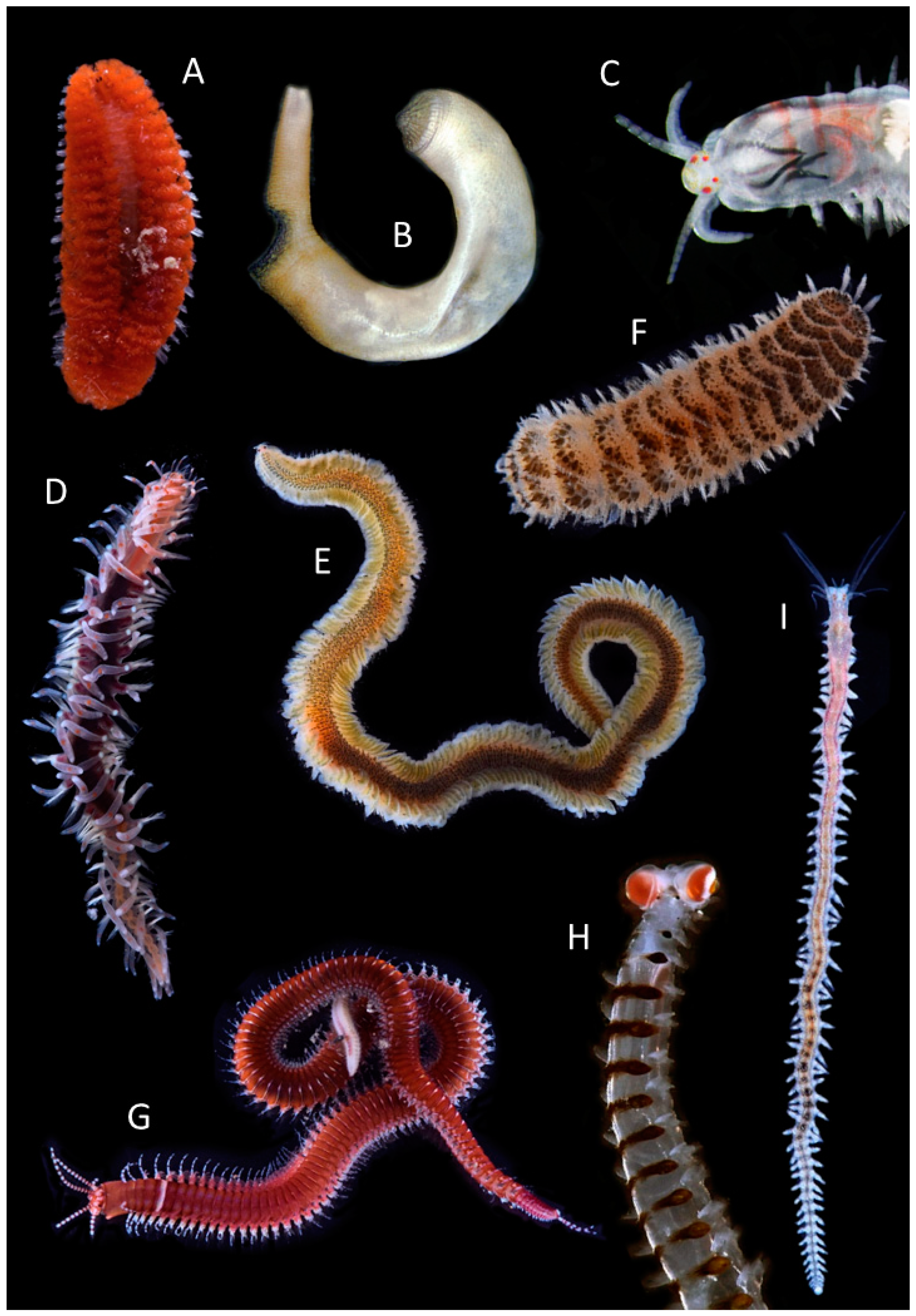This photograph displays a diverse collection of organisms labeled A to I, against a solid black background. Each organism is distinct in appearance, often resembling worms, centipedes, or millipedes, with various invertebrate features.

- **A**: Resembles a pair of bright red lips, adorned with white furs around its edges.
- **B**: Appears worm-like, possessing a white and brown segmented body, curled into the shape of the letter C. 
- **C**: A white organism accented with red stripes, featuring two white antennae and patterned with red and yellow dots on its face.
- **D**: Another worm-like creature, colored red with long white fibers extending from its body.
- **E**: A longer worm, brown with tan and white fibers, similar in texture to D.
- **F**: Stockier and shorter, brown in color interspersed with darker brown dots and short white fibers.
- **G**: This longer worm is bright red, covered similarly with white fibers, closely resembling millipedes.
- **H**: Extending off the page, this clear worm-like creature has brown lines and distinctive white eyes.
- **I**: The longest worm, characterized by its white and brown dotted body, adorned with white fibers and antennae.

The highly detailed image captures these segmented and often translucent creatures, highlighting their unique physical traits and wide array of colors.